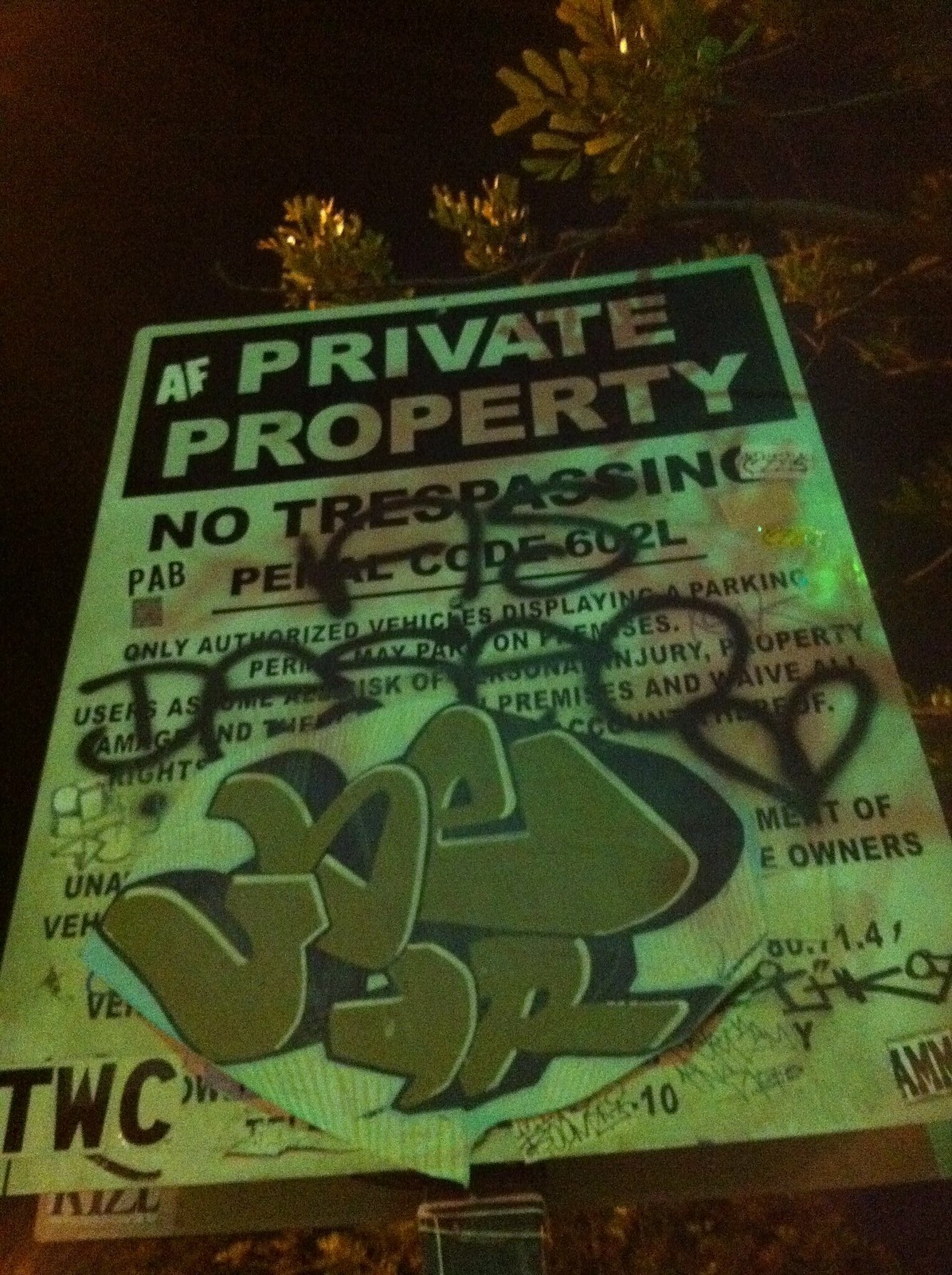This detailed photograph, captured at night, predominantly features a defaced "Private Property" sign. The sign, centered in the lower two-thirds of the vertical rectangular image, stands out against a particularly dark background where faint outlines of tree branches and leaves are visible, contributing to a yellowish hue cast over the scene.

At the top of the sign, within a black rectangle, the bold white letters read "PRIVATE PROPERTY." Below this, though partially obscured by extensive graffiti, the text states "NO TRESPASSING," followed by the penal code "602L." Further down, additional instructions specify that only authorized vehicles with a parking permit may park on the premises, although this section, much like the rest of the sign, has been heavily defaced.

Various forms of defacement obscure the sign, including black spray paint, green graffiti, and other markings. There's a hole in the sign filled with some substance, adding to its aged and neglected appearance. The lower left corner of the sign shows large black letters "TWC," and the lower right includes a symbol resembling "OKG." The overall decay, with visible dirt and mold, suggests the sign has been exposed to the elements for a significant time. The scene, shrouded in darkness, and the vandalized sign collectively create a somber, eerie atmosphere.